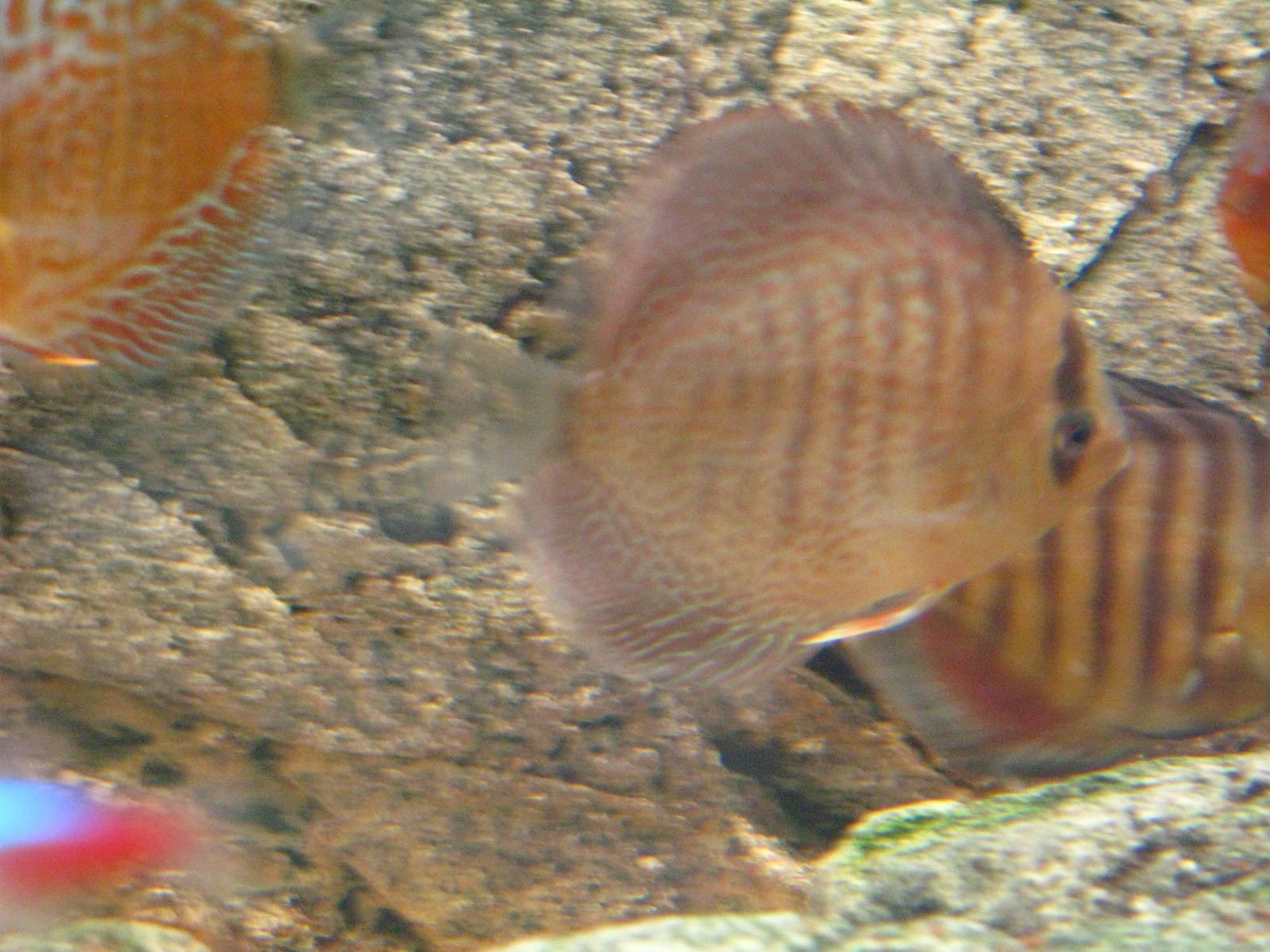The image is a large, slightly blurry photograph of an aquarium with a rocky, light gray to tan background, some rocks having patches of green moss. The bottom of the aquarium is covered in pale stonework, and multiple colorful fish populate the scene. On the left bottom corner, there's a fish with a light blue top and a pinkish-red underside. In the upper left corner, an orange fish with faint orangish gills and an orange and white pattern is partially visible. The centerpiece of the image is a fish with a round, flattened body and a striking pattern of black vertical stripes across its brown body, adorned with red dots. This fish, which has prominent fins along its top and bottom, sports a wider black vertical line at the front near its black eye. Underneath this central fish, another fish with black vertical stripes and mostly orange gills can be seen. In the upper right corner, a faint glimpse of an orangish fish swimming away is visible. The overall scene, slightly out of focus, captures the dynamic and colorful essence of an aquarium environment.